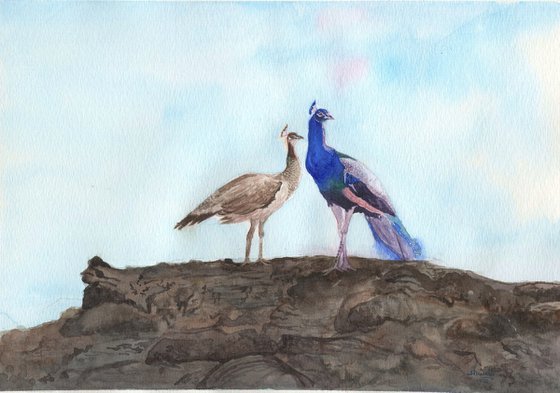This detailed drawing, potentially created using pencil, watercolor, or digital techniques, showcases two peacocks standing on a brown, rocky structure against a backdrop of a blue sky adorned with subtle, light clouds. The male peacock, positioned on the left, exhibits a vibrant blue crest and head, transitioning to a greenish hue toward the body, which also features white, black, and bluish undertones extending to the tail. The female peacock, smaller and positioned to the right, displays a predominantly brown and gray coloration, with a darker gray head and crest. The artwork is signed in black in the lower left corner, though the signature is indistinct. The overall composition captures the striking contrasts between the richly colored male and the more subdued female, enhancing the natural beauty of these elegant birds.